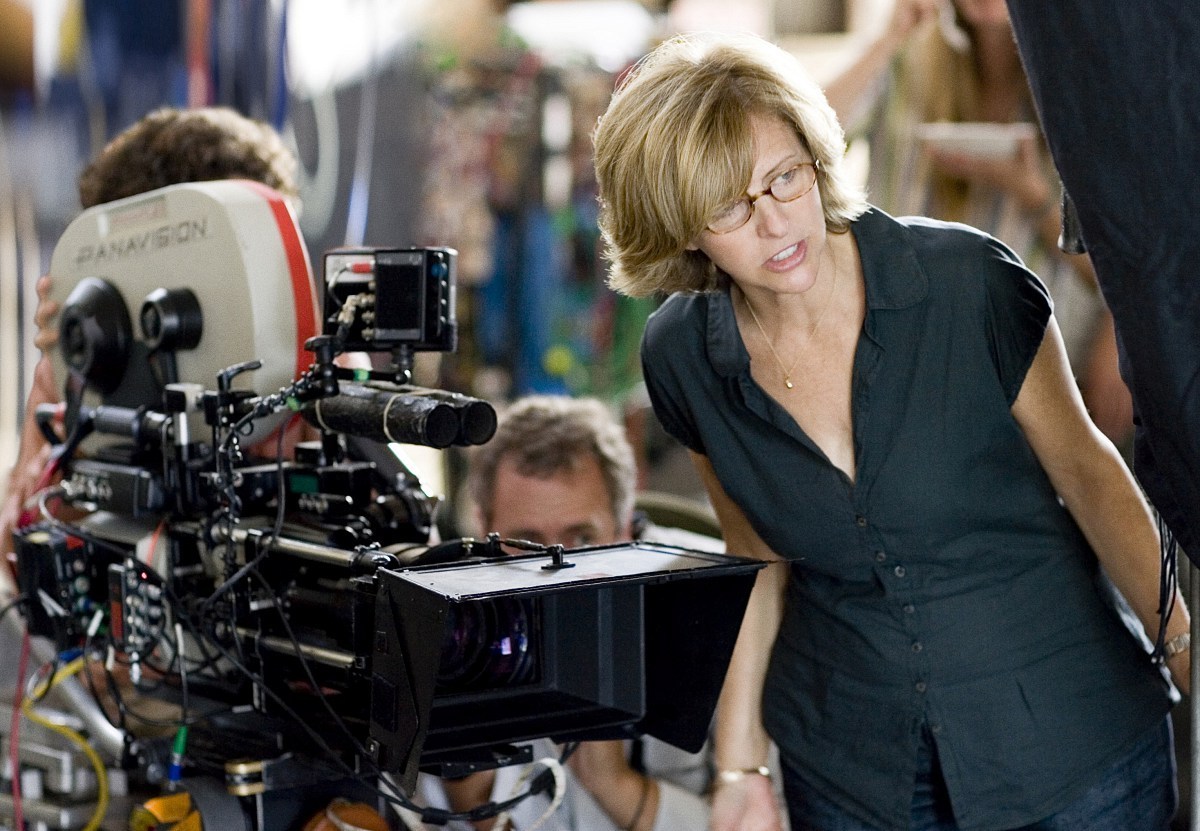The image captures a detailed, busy scene on a film set. Central to the image is a technically advanced Panavision camera with intricate features resembling small telescopes, marked prominently in white and red. Positioned on the left side, the camera is surrounded by wires and instrumentation, adding to its complexity.

To the right, a short-haired blonde woman is intently peering into the camera's viewfinder to match its angle, suggesting she is directing the film. She wears a black v-neck blouse buttoned to her chest, with a necklace and bracelets visible. Her glasses rest low on her nose as she focuses on the shot.

Behind the camera, a man with only his hair visible and partially obscured by the equipment, holds the camera’s right side. Next to him, partially hidden and slightly to the right, is a second man with curly, balding hair, visible only by his eyebrows and one eye, with one hand showing beneath the camera.

The background of the scene is blurred, emphasizing the intense concentration of the people involved in the filmmaking process. This detailed snapshot captures the coordinated efforts of the directing and camerawork teams in action.